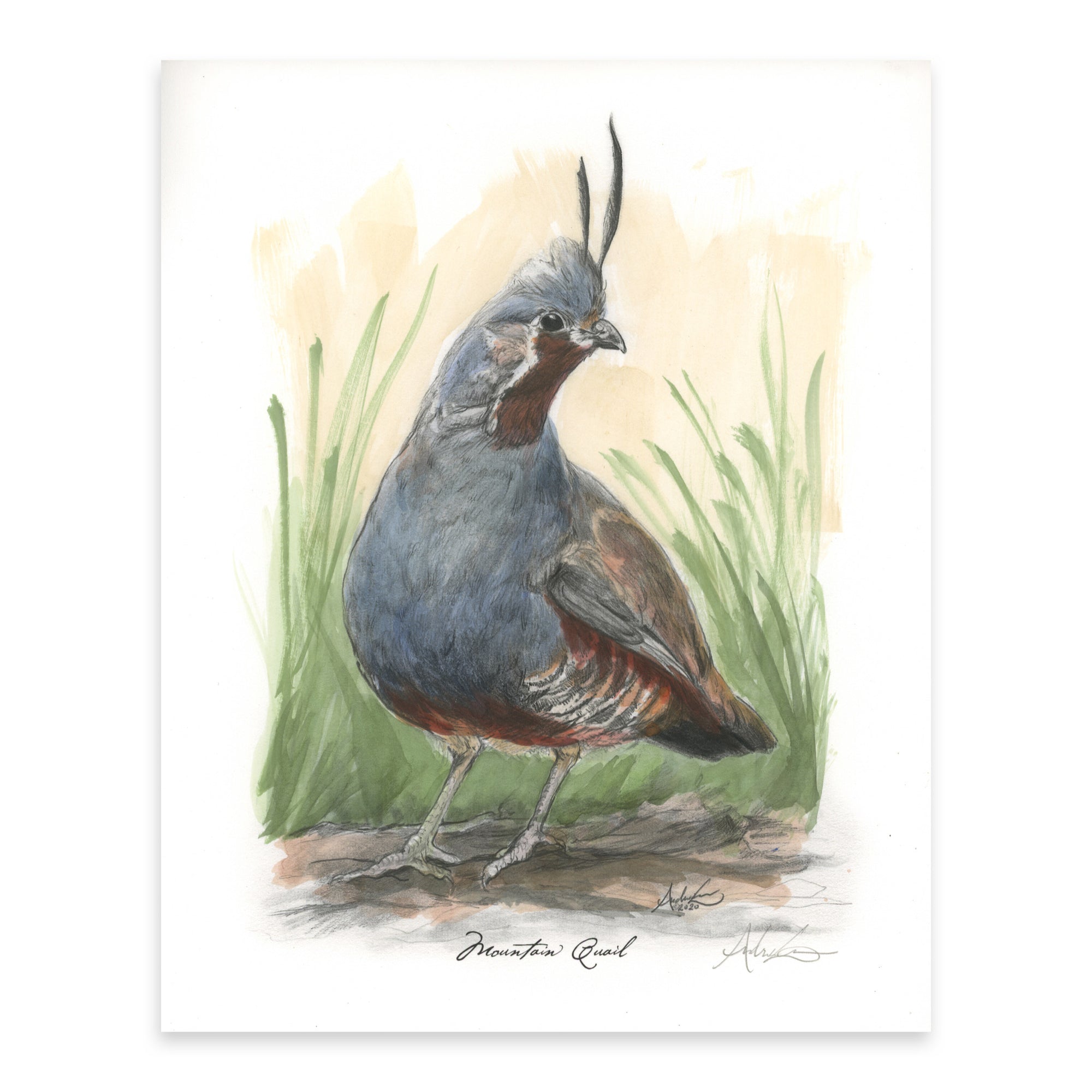This image displays a detailed painting of a Mountain Quail, prominently placed against a white canvas or paper background with a slightly folded upper-left corner. The quail stands on a brownish-gray rocky ground, exhibiting shadows beneath it for depth. Behind the bird, primitive streaks of green hint at grass and plant life, combined with tan and light brown shades to enrich the background. 

The quail itself is depicted with a predominantly gray body, including the forehead, neck, upper body, and belly. Its throat region is a distinct brown, matching the shades found on its wings and tail. The bird features two distinctive feather plumes atop its head, black eyes, a small sharp beak, and brown legs. 

The painting includes the title "Mountain Quail" written in a black cursive script at the bottom. Interestingly, the artist has signed the piece twice in different locations, with both signatures beginning with the letter 'A'. The quail's head is turned to the right side of the picture while its body faces left, capturing a moment of poised alertness.